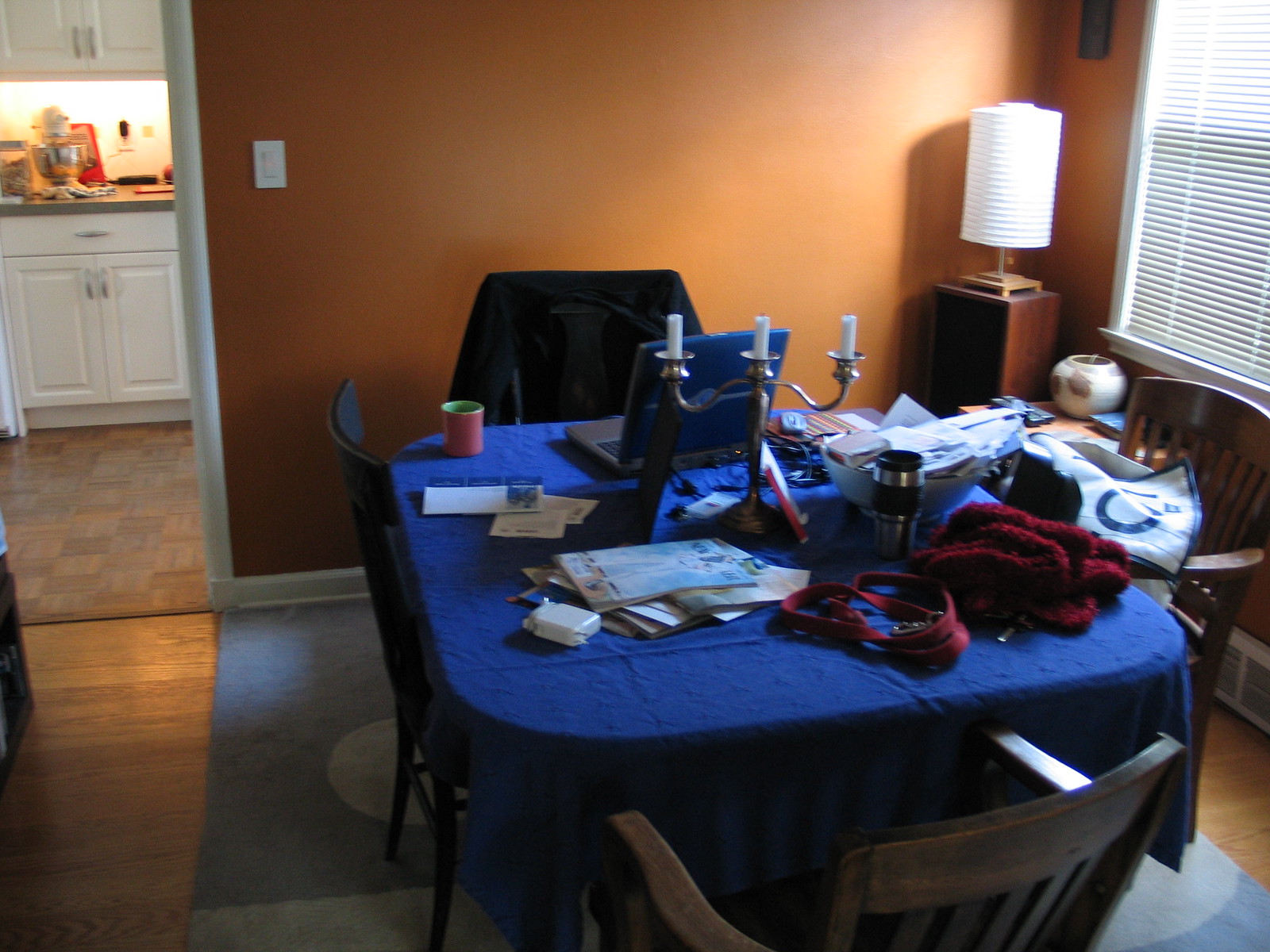In the image, the background features a brown wall equipped with a white light switch. On the extreme right edge, partially drawn blinds allow light to filter through the top. A lamp with a white fabric shade sits on a brown square base, casting light into the room. Below it, a table covered in blue fabric is visible, accompanied by red fabric and what appears to be a red leash with a metal hook resting in the bottom right corner. 

On the left-hand side of the table lies a pile of papers, and in the center stands a candelabra holding three white candles, their wicks unlit. A chair on the right side has a piece of fabric draped over it, while another chair at the far end of the room bears a casually placed shirt. Nearby, a pink mug with a green interior and a laptop with a blue backing and keyboard are placed atop a surface.

Towards the far left, the image extends into a kitchen with a wood-tiled floor. The kitchen area is well-lit, showing a bowl, possibly a mixing bowl, situated at the back end along with a drawer at the bottom and an open cabinet door up top. The main room is adorned with a large rug featuring a pattern of blue and white squares.